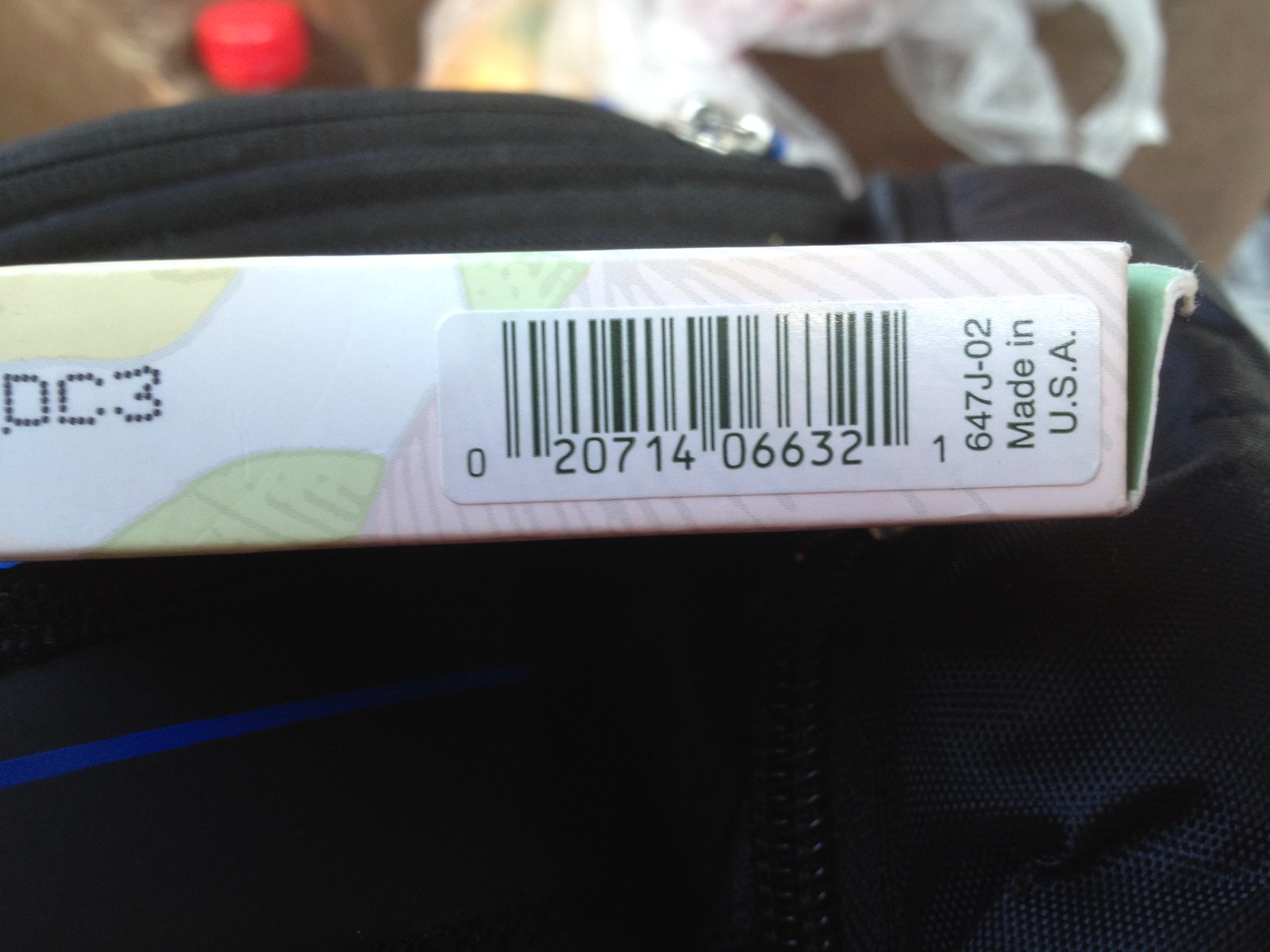This photograph captures a detailed view of a packaged item resting on a black zippered surface, which appears to be part of a backpack. The black backpack is prominently featured with a silver zipper and a distinctive blue stripe towards the bottom edge of the image. The packaging itself is predominantly light pink, adorned with a green leafy design, and features a barcode accompanied by numbers underneath. The text "647J-02, Made in USA" is printed in black font at the bottom of the package. In the background, besides the backpack, a red lid and a glimpse of a plastic bag are visible, adding context to the setting. The various elements combine to create a visually rich and descriptive scene.